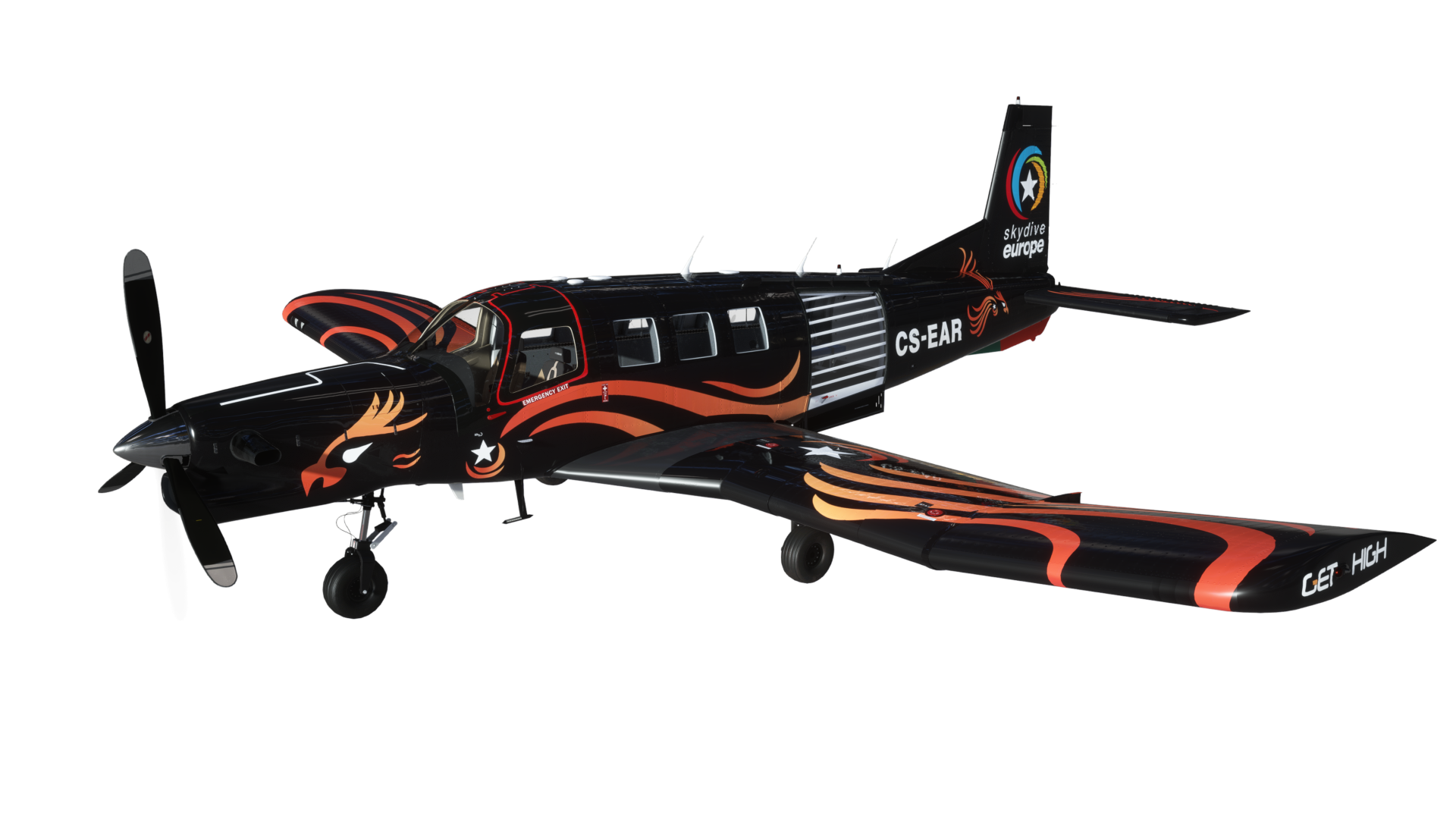The computer-animated image features a small, single-engine trainer aircraft prominently displayed against a white background. The aircraft's body and wings are primarily black, adorned with a striking pattern of red, yellow, and white stripes. Distinctively marked with the identifier "CS-EAR" in bold capital letters, the plane also boasts a colorful emblem reading "Sky, Europe" alongside a prominent white star logo. An artistic depiction of an eagle with an orange beak and light orange feathers is beautifully integrated into the design, adding an extra layer of visual appeal. The wings bear additional orange stripes and the motivational phrase “Get High,” further emphasizing the aircraft's dynamic nature. There are two visible wheels situated at the bottom, and the overall design includes detailed features such as a propeller with black and silver-tipped blades, and four windows, including the pilot's. The detailed motifs and functional aesthetics suggest that this multi-role utility workhorse is well-suited for both training and skydiving operations, potentially within a simulated environment.